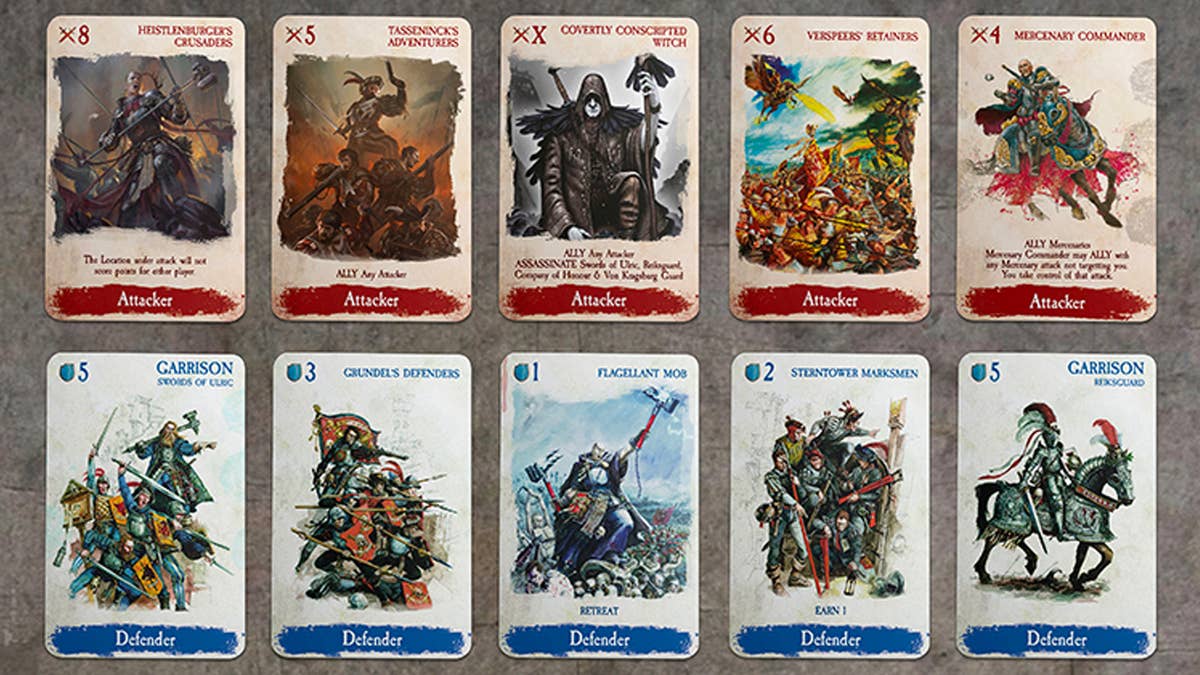This photograph showcases 12 playing cards from the Warhammer Fantasy card game, arranged in two rows of six on a gray background. The top row features attacker cards, identifiable by their tan and red color scheme, with a red paint stroke at the bottom bearing white text that reads "attacker." Each attacker card also displays an illustration of a character engaged in combat, such as people with swords and mythological creatures like horses and dragons. In the upper left corner of these cards are numerical values, and a pair of crossed swords icon, while the character names are situated in the upper right corner. Beneath the illustrations, there are descriptions of the actions that occur when the card is played. The bottom row consists of defender cards, highlighted by a blue paint stroke with white text that reads "defender." These cards also feature character illustrations, including a knight on a horse with armor. The upper left corner of each defender card displays a blue shield icon alongside a numerical value. This detailed arrangement and the visual elements distinctly segregate the attacker and defender functionalities within the game.